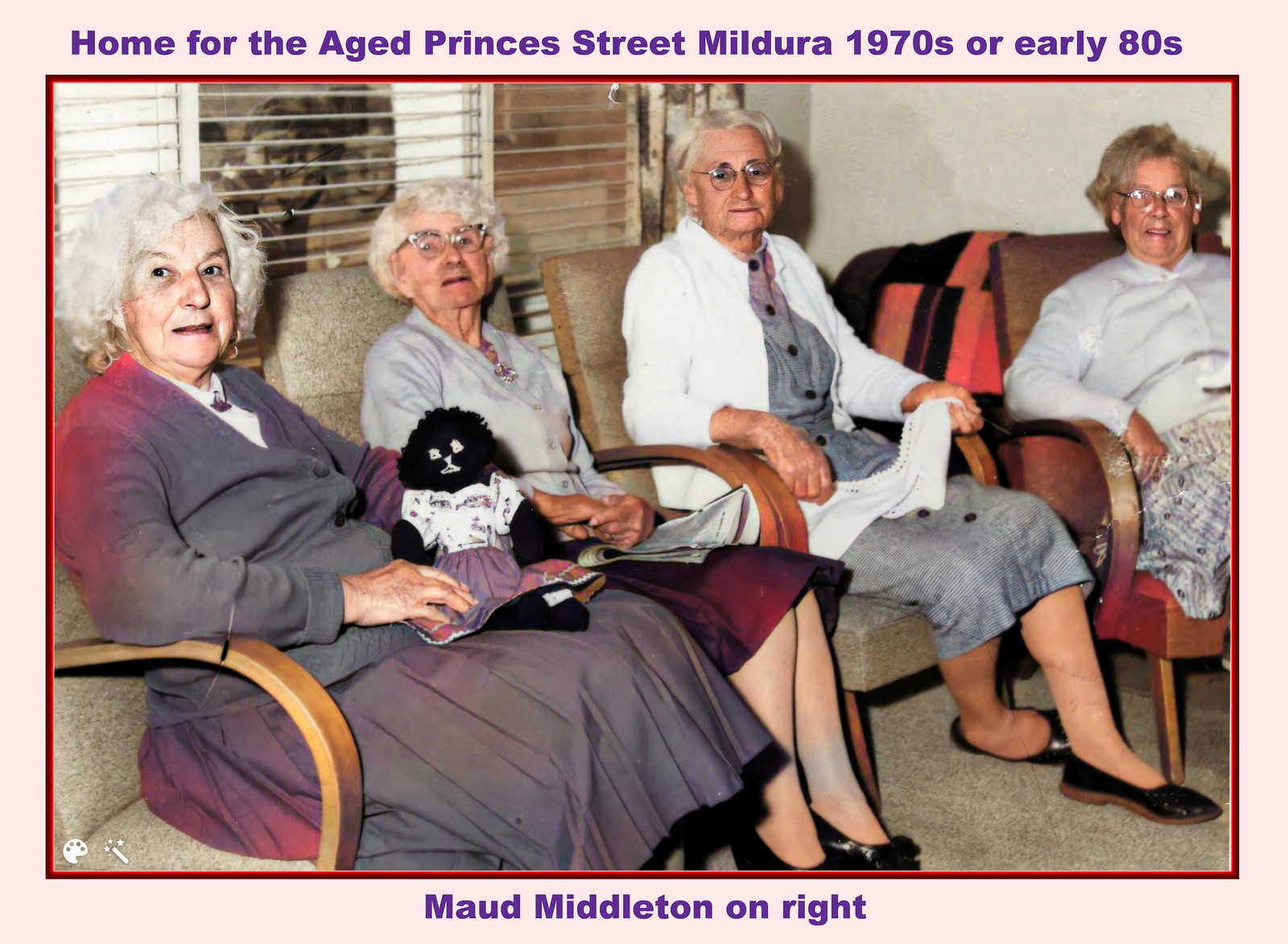This detailed photograph showcases four Caucasian senior women with white hair, seated in a row of individual wooden chairs in a room with white walls and beige carpet. Each woman is dressed in distinctive attire. From left to right, the first woman wears a gray long-sleeved sweater with a matching skirt and has a doll in a dress sitting on her lap, her right arm resting on the chair's arm. To her left, the second woman dons a gray button-up sweater, cat-eye glasses, a red knee-length skirt, and black shoes with stockings. The third woman sports a white button-up sweater over a gray dress, glasses, black shoes, and has her left leg crossed over her right while holding a handkerchief or knitting in her left hand. The fourth woman wears a white sweater buttoned to the neck, glasses, a patterned skirt, and her right arm rests on the chair's wooden arm. The background features open Venetian blinds on the windows and an Afghan or blanket can be seen hanging. Above the image, in the light pink border, purple text reads "Home for the Aged Prince's Street Mildura 1970s or early 80s," and the subhead at the bottom reads "Maud Middleton on right." The photograph, rendered in a style combining photographic realism with graphic design, captures a moment of serene camaraderie among the elderly women.